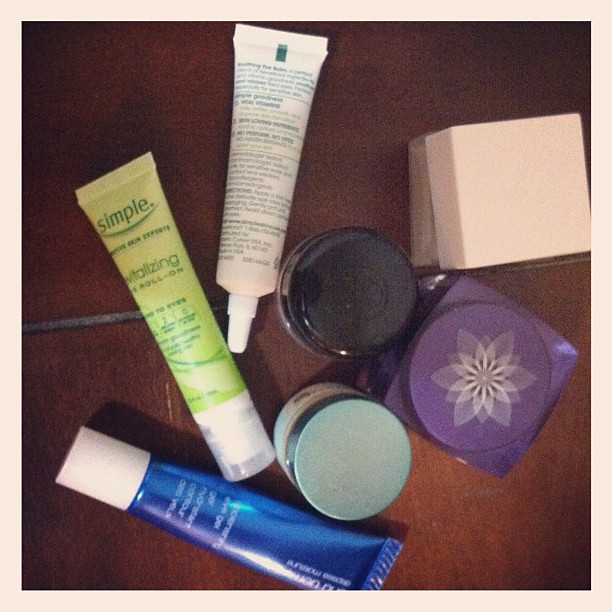This image showcases an array of makeup products and skincare items, all neatly arranged on a brown wooden table. The wooden surface has a visible seam running through its middle. 

Starting from the bottom of the image, there's a long blue tube with an unreadable label and a white cap. Above and to the left is a greenish-yellow tube labeled "Simple," partially readable with the words "vitalizing" and "roll on," topped with a clear lid that seems to house a pump inside. 

Further up, there's a smaller white tube viewed from the back, featuring a white, fine tip and extensive writing. To the right of these tubes are two circular containers: the first one, likely a pressed powder, has a dark lid, while the second, positioned beneath it in the image, has a blue lid with a white base, possibly containing face cream.

Adjacent to these, on the right, is a purple square container decorated with a white flower on top, potentially holding bath beads or lotion. Above this item, there's another square container with a solid peach lid and an opaque base of the same color.